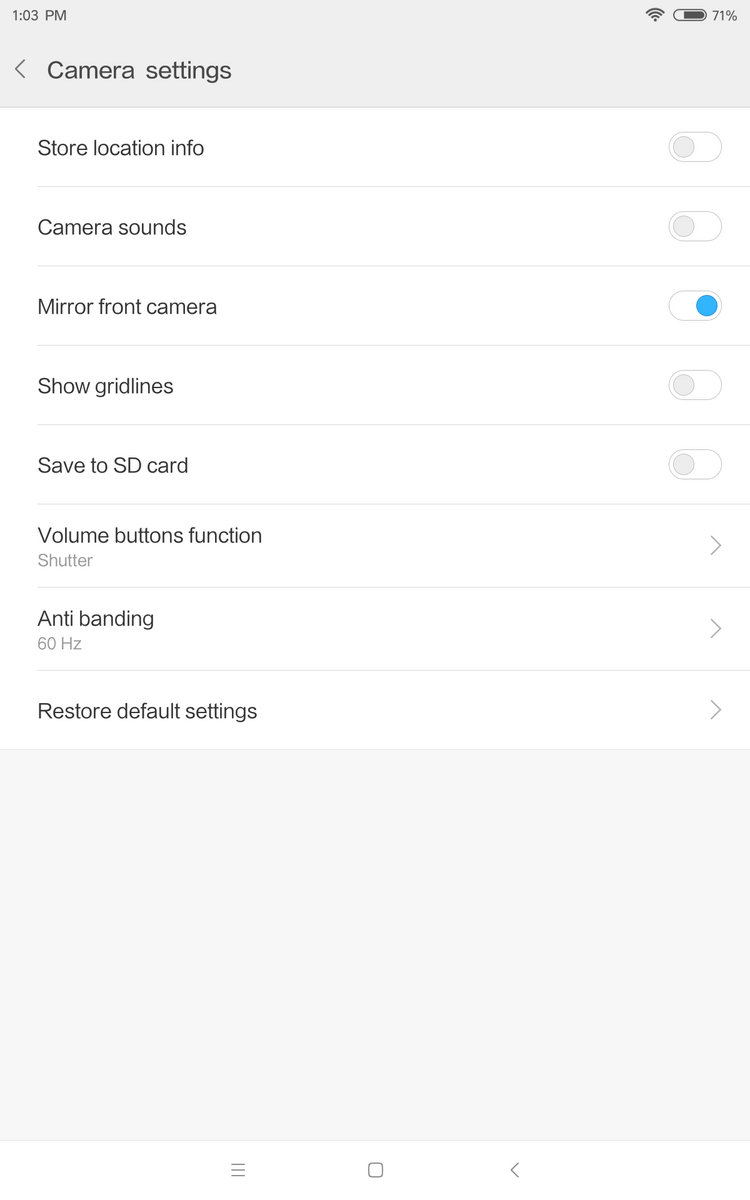The image displays a screenshot of a smartphone's camera settings. The timestamp on the phone reads 1:03 PM, and the battery indicator shows 71% remaining. In the settings menu, the option "Mirror Front Camera" is visibly toggled on. Other options such as "Store Location Information," "Camera Sounds," and "Save to SD Card" are turned off, evident by their unchecked boxes. The user seems to have specifically accessed the settings to ensure that the "Mirror Front Camera" feature was enabled. The overall layout of the screenshot is clean, highlighting the primary focus on camera configuration options.